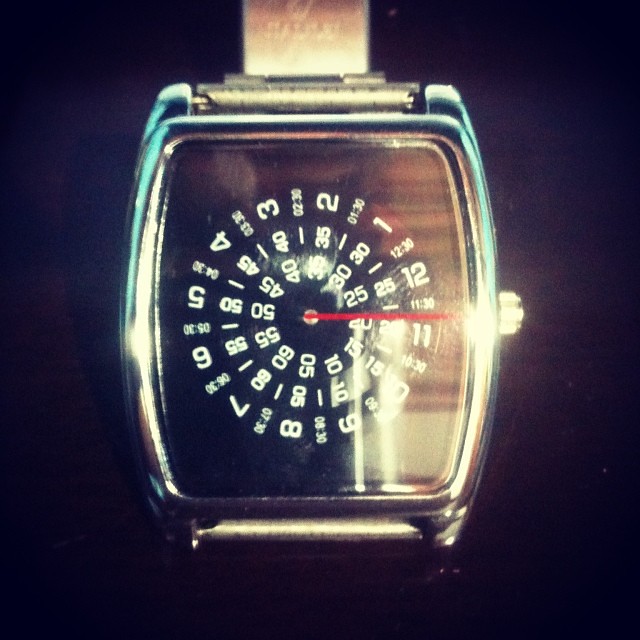This image features a unique wristwatch with a distinctive design. The photograph itself appears to be of lower quality, possibly an older image. The wristwatch stands out due to its unusual arrangement of numbers on the face. The numbers, starting from 1, follow a swirling circular pattern that arches and gradually tightens, eventually reaching up to 60. As the numbers spiral inward, the font size decreases, adding to the intricate aesthetic. The watch has a single red ticker hand that contrasts with the face, which has a wooden texture as its backdrop. Encasing the face is a square, silver frame, further emphasizing the watch's unique and artistic design.